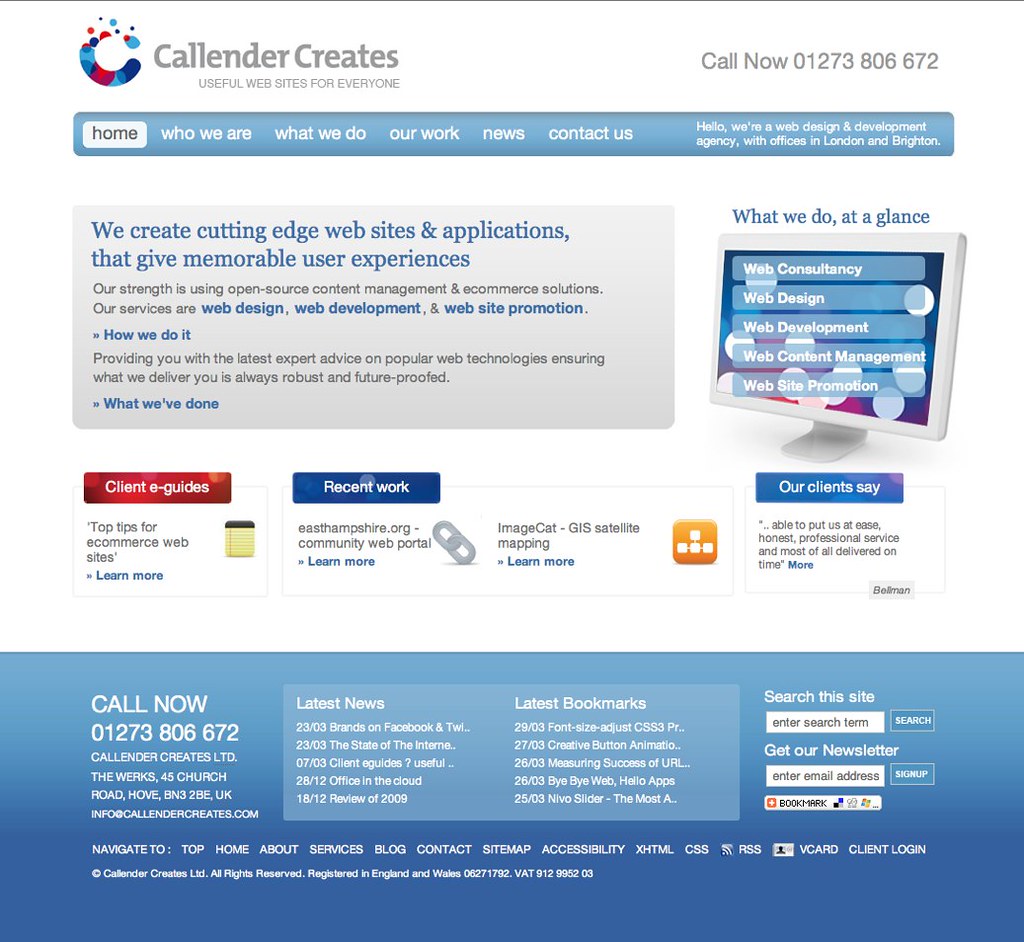**Calendar Creates Website Overview**

**Contact Information:**
- **Company Name:** Calendar Creates
- **Location:** The Weeks, 45 Church Road, Hove, BN3 2BE, UK
- **Phone Number:** 01273 806672
- **Email:** info@calendarcreates.com

**Website Navigation:**
- **Main Sections:** Home, Who Are We, What Do We Do, Our Work, News, Contact Us

**Services Offered:**
- **Web Consultancy:** Expert advice on popular web technologies, ensuring robust and future-proof solutions.
- **Web Design:** Creating cutting-edge websites with memorable user experiences.
- **Web Development:** Building applications using open-source content management and e-commerce solutions.
- **Web Content Management:** Organizing and managing website content efficiently.
- **Website Promotion:** Strategies to enhance online presence and visibility.

**Detailed Description:**
Calendar Creates specializes in crafting innovative websites and web applications that provide memorable user experiences. Utilizing cutting-edge technologies and open-source solutions, they offer comprehensive services including web consultancy, design, development, content management, and promotion. Their expert team ensures that each project is future-proof and tailored to client needs.

**Portfolio Highlights:**
- **Showcased Work:** Examples include easthampshire.org and the imagecat GIS satellite mapping web portal.
- **Client Testimonials:** Positive feedback highlighting effective service and delivery.
- **Guides and Tips:** E-guides and top tips for e-commerce websites.

**Footer Information and Additional Features:**
- **Contact Details Reiteration:** Phone: 01273 806672 | Address: The Weeks, 45 Church Road, Hove, BN3 2BE, UK | Email: info@calendarcreates.com
- **Social Media:** Links to example brands on Twitter and Facebook
- **Latest Bookmark:** Font size adjust CSS3 property
- **Newsletter Sign-Up:** Option to enter email address for updates
- **Quick Links:** Home, About, Services, Blog, Contact, Sitemap, XHTML, CSS, RSS, vCard, Client Login

This detailed summary encapsulates the services, contact information, and significant sections highlighted on the Calendar Creates website, offering a comprehensive overview of what they offer and how they engage with clients.